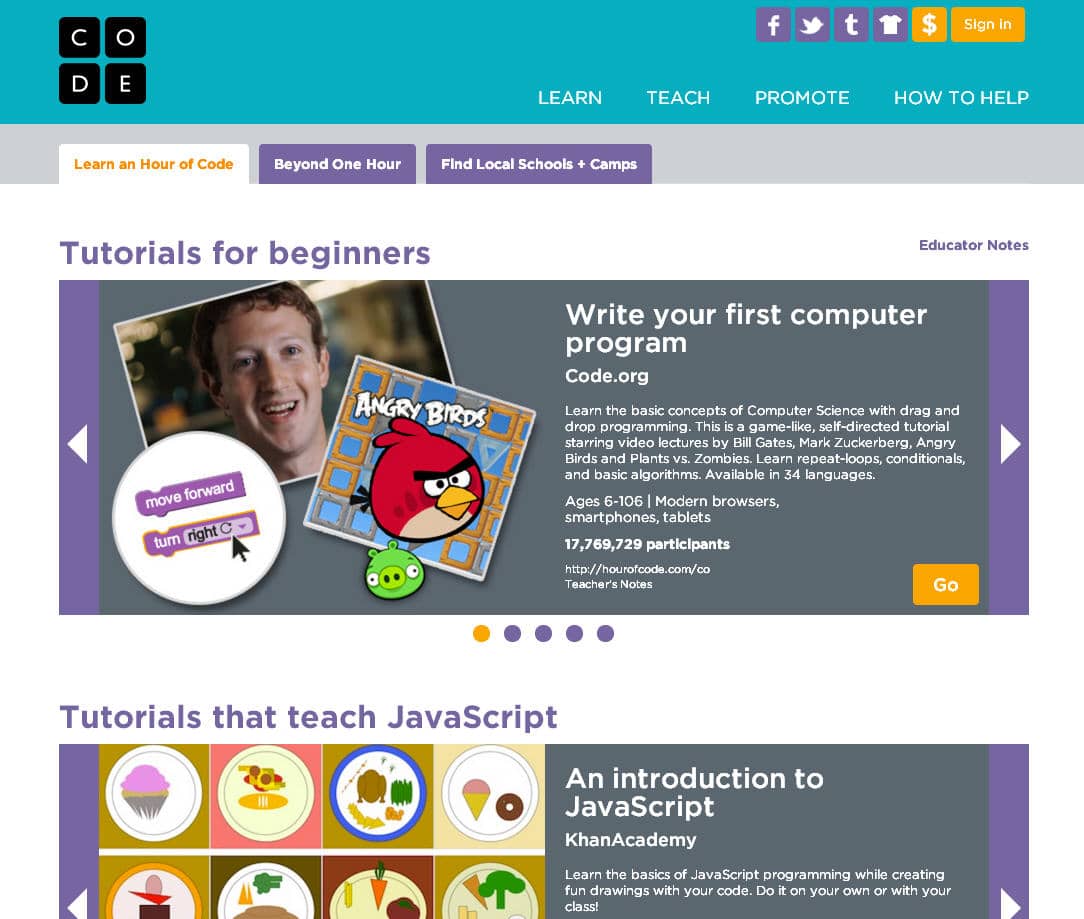In this screenshot of a coding website, the upper left-hand corner features four black squares, each containing a letter that collectively spell out "CODE." On the right side, the options "LEARN," "TEACH," "PROMOTE," and "HOW TO HELP" are displayed alongside icons for Facebook, the old Twitter, Tumblr, a t-shirt, a dollar sign, and a "SIGN IN" button.

The main navigation includes tabs labeled "LEARN AN HOUR OF CODE," "BEYOND ONE HOUR," and "FIND LOCAL SCHOOLS PLUS CAMPS." The "LEARN AN HOUR OF CODE" tab is currently selected, revealing a section titled "TUTORIALS FOR BEGINNERS." This section invites users to "WRITE YOUR FIRST COMPUTER PROGRAM" via CODE.org and promises to teach the basic concepts of computer science using drag-and-drop programming. It touts a self-directed tutorial featuring video lectures by notable figures such as Bill Gates and Mark Zuckerberg, as well as characters from "Angry Birds" and "Plants vs. Zombies."

The tutorial aims to teach concepts like repeat loops, conditionals, and basic algorithms, and is available in 34 languages for users aged 6 to 106. Beneath this, another section highlights "TUTORIALS THAT TEACH JAVASCRIPT," offering an introduction to JavaScript by Khan Academy. Users can learn the basics of JavaScript programming while creating fun drawings with their code, either independently or as part of a class.